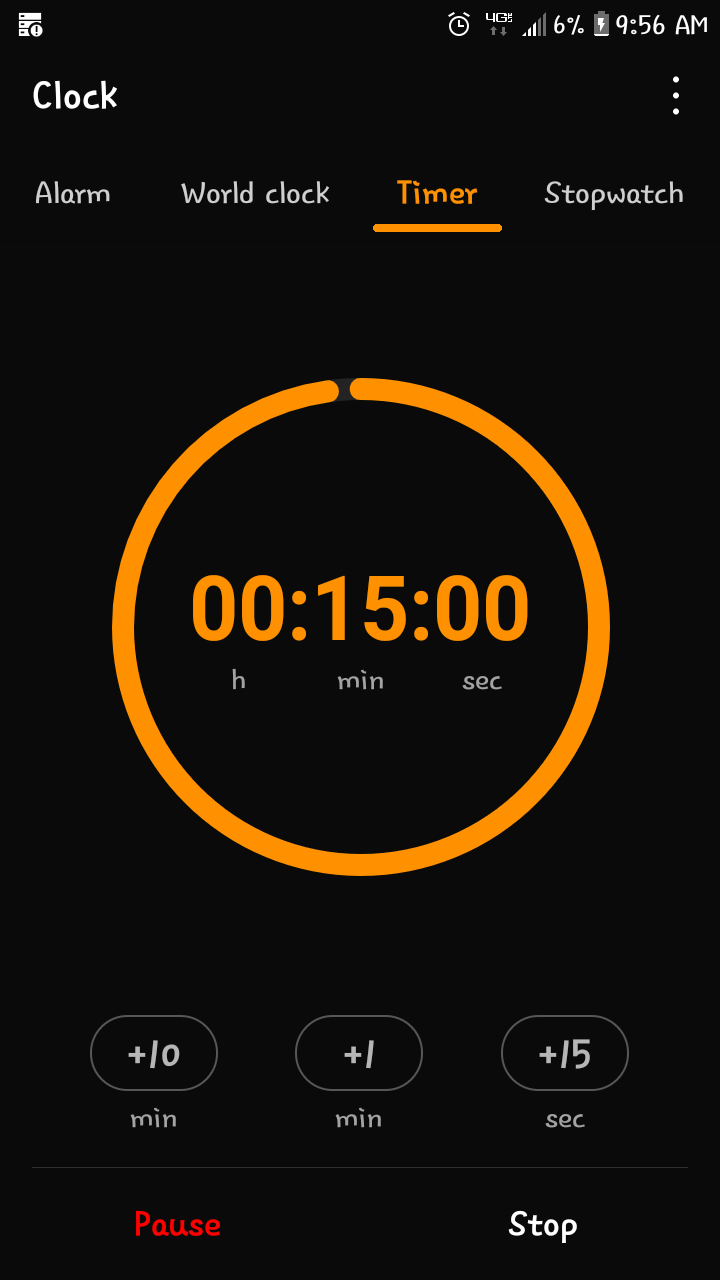The image depicts a clock interface on a mobile screen with a predominantly black background. At the top of the screen, "Clock" is displayed in white text. In the top-right corner, typical status indicators show that the battery life is at six percent and currently charging, indicated by a lightning bolt within the battery icon. The current time is 9:56 a.m. Directly underneath, there are three dots that likely lead to the settings menu.

The interface is currently on the "Timer" tab, the third of four available sections, with the other options being Alarm, World Clock, and Stopwatch. The Timer tab is highlighted in orange with an underline beneath it. In the timer section, a countdown is set for 15 minutes (0 hours, 15 minutes, 0 seconds) and is encircled by a blue progress indicator, suggesting that pressing play will start the countdown, reducing the blue circle over time.

Below the timer display, there are two sets of minute adjustment tabs and one for seconds, which allow for incrementing or decrementing the time. The play button is distinctively marked in red, while the stop button is in white.

A handwritten, informal font style is used throughout the interface, lending a casual and unique aesthetic to the display. The letters, particularly "A," appear to be cool and almost hand-drawn, diverging from more formal digital fonts.